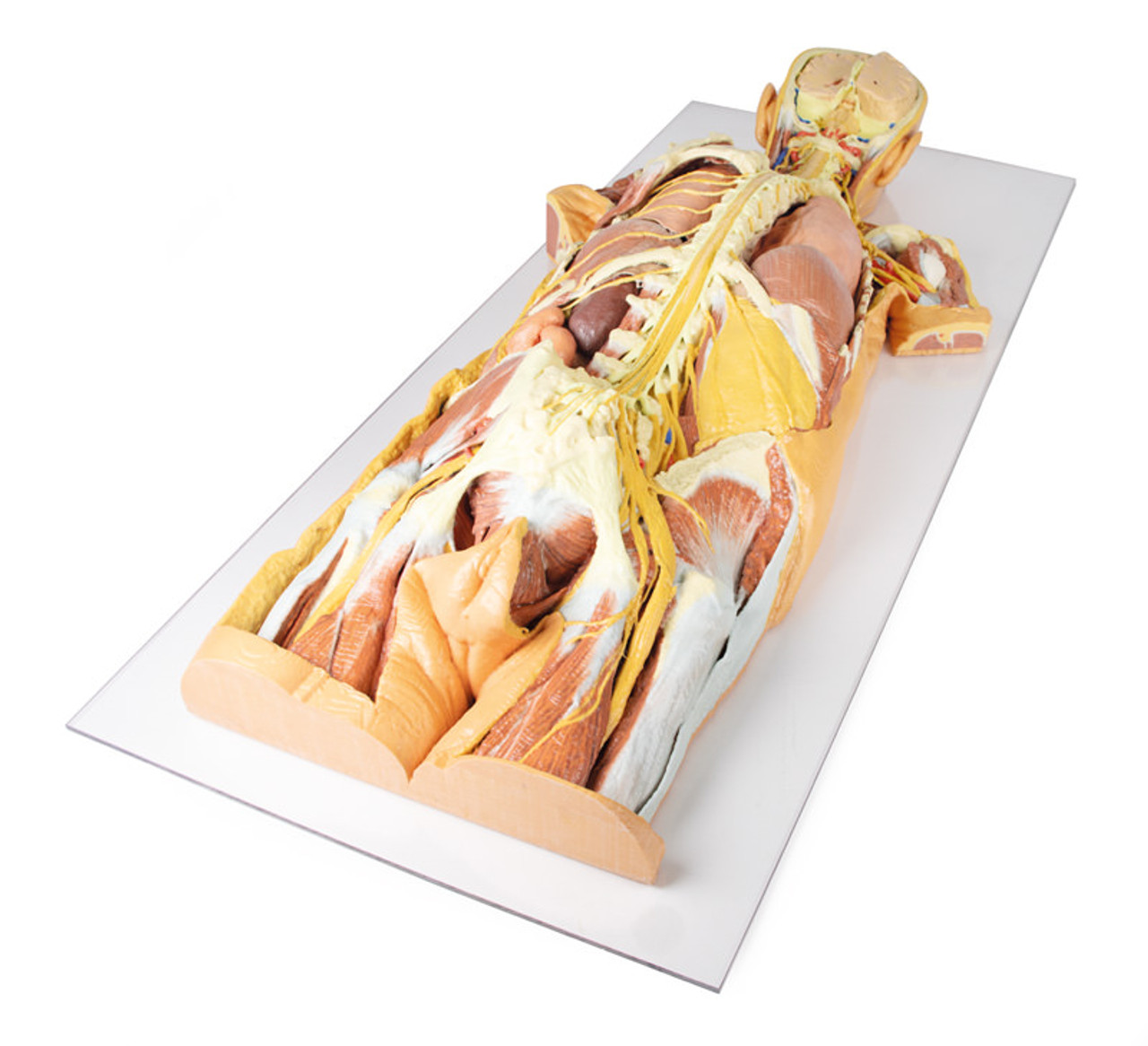The vertical, borderless image depicts a partially dissected human cadaver lying face down on a flat white rectangular surface. The body, with blondish hair, has had most of its skin removed, revealing intricate muscles, bones, and internal organs. The arms are severed at the shoulders, exposing the shoulder joints, while the legs are cut off at the lower thigh, leaving visible thigh muscles and bones. The detailed view includes the spine, hip bones, and leg bones, along with prominent organs such as the lungs, liver, and kidneys. The back of the head is open, displaying the brain partly covered by the skull cap, and the ears are visible, suggesting the subject might be an older individual. The dissection is thorough, allowing a view of the red fibrous muscles, white ligament material, the bowels, and even the remaining skin around the anus.